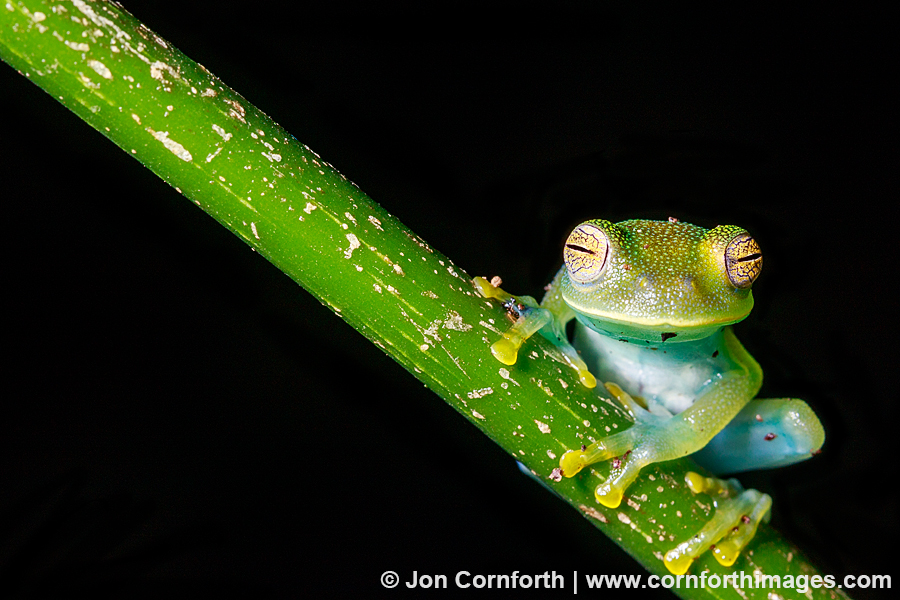This is a high-definition color photograph, depicting a vivid close-up of a tiny, bright lime-green frog perched on a similarly green stem of a plant, set against a completely black background. The frog, exhibiting remarkable camouflage, faces the camera and is located in the lower right section of the image, specifically on the diagonal stem that spans from the upper left to the lower right corner. The frog’s eyes, which are tiny slits and almost closed, showcase a unique yellow hue with black slit pupils. The frog also has a few small tan spots on its head and tan-colored streaks within the stem, adding subtle contrast. Additionally, the frog’s belly and chin are a stark white, providing a strong visual contrast to its bright green body and partially yellow-tinted legs. In the lower right corner of the photograph, the white text attribution reads "© John Cornforth | www.cornforthimages.com."